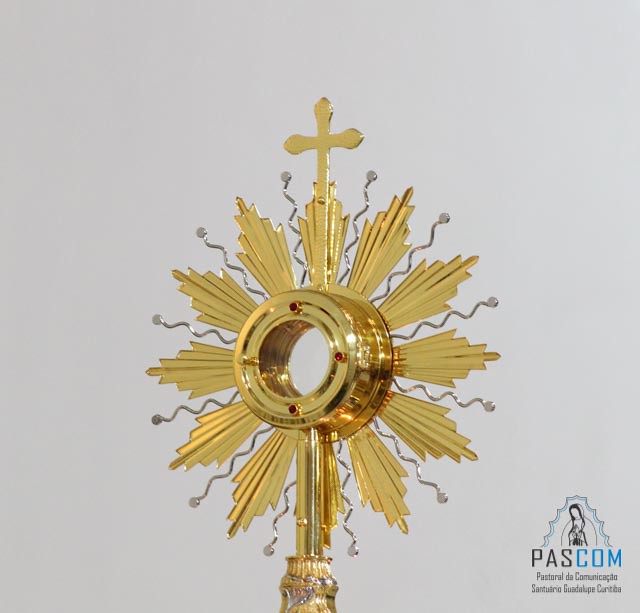This square image depicts a highly detailed, ornate gold medallion that is likely used in religious ceremonies. The medallion, which is bright and shiny, sits atop a golden decorative pole or staff, suggesting its significance in a high-ranking religious context. It features a central, circular area with petal-like protrusions and a hollow middle, allowing a view of the uniform gray background behind it. Between the petals are zigzagging lines that add to the intricate design. Notably, there are red jewels studded in three quadrants of the circle, while the fourth quadrant hosts a gold jewel. Emanating from the center in a circular pattern are golden rays, giving it a sunburst appearance. At the very top of this radiant design is a small gold cross, crowning the medallion. The image also includes a logo in the bottom right corner that reads "PASCOM" along with text too small to discern clearly, and possibly an image of the Virgin Mary. The decorative nature and the detailed workmanship of this medallion underscore its ceremonial importance.